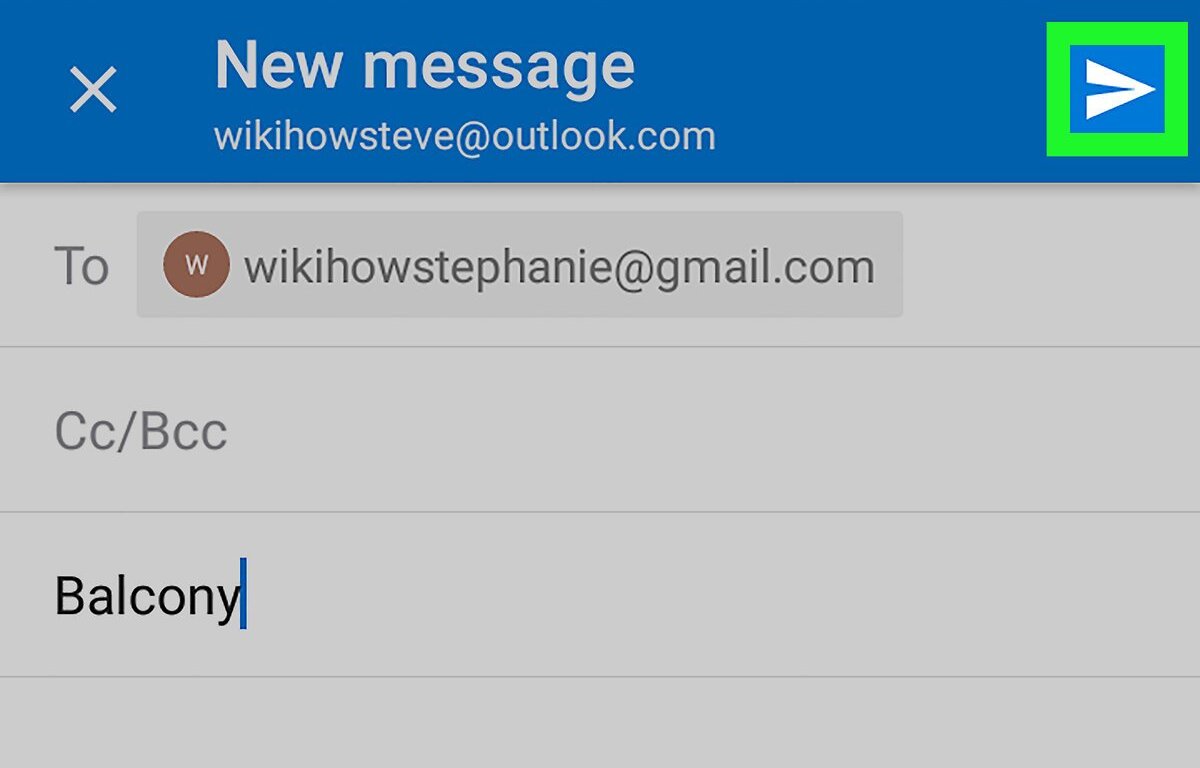This image depicts a screenshot of an email interface. The header is a medium shade of blue and features several elements: a white 'X' icon positioned on the left, followed by the words "New Message" written in bold white text. Directly beneath this, in smaller white text, is the email address "wikiHowSteve@Outlook.com". In the upper right corner of the header, there is a logo consisting of a neon green box with a smaller blue box inside it, and a triangular white shape at the center.

Below the header, there are four gray lines. The first line includes the label "To:" followed by "wikiHowStephanie@Gmail.com" and is accompanied by a brown circle with a white 'W' to the left of the email address. On the left side of the second line, the text "Cc/Bcc" is visible. Beneath these lines, in black text, the word "Balcony" is displayed.